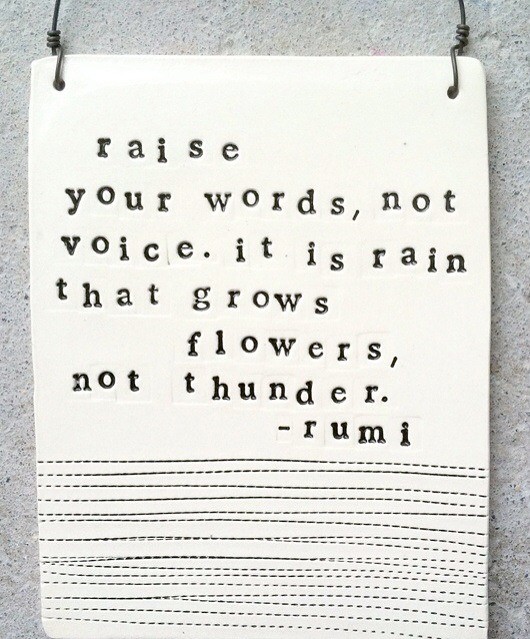The image displays a tall, rectangular sign made of an off-white, ceramic-like material. It hangs slightly askew against a textured gray wall, suspended by dark wires threaded through holes in the top left and right corners, which are cut off at the top of the image. The sign itself is gently curved along its sides. Engraved in unevenly placed black letters, it reads: "raise your words, not voice. it is rain that grows flowers, not thunder. - rumi." Below the quote, the sign features several horizontal stripes of dotted lines, numbering at least sixteen. This quaint and meaningful sign serves as an elegant reminder when hung on a wall.